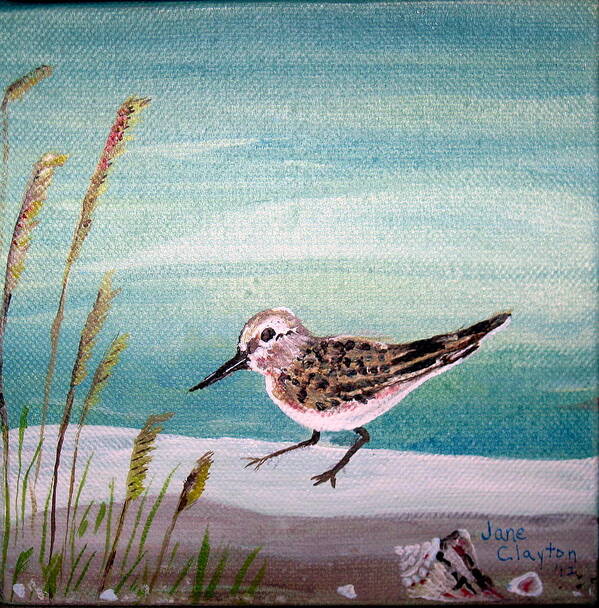This detailed painting by Jane Clayton depicts a bird standing at the shoreline, surrounded by elements of nature. The bird, central in the lower half of the square canvas, faces left with a distinctive black beak pointed downward. Its gray and white face contrasts with its dark, speckled brown and black body, and it has a white belly, dark legs, and toes. The bird's dark tail features fine black lines.

The background, painted in shades of blue, light green, and white, suggests waves or a sky that covers the upper two-thirds of the image. Tall, waving seagrass with green stalks, yellow tips, and occasional red highlights frames the left side of the scene. The ground beneath the bird is divided into two sections: a white strip above a reddish-brown base. Scattered in the bottom right corner, there's a large white seashell with black and red highlights, accompanied by smaller shells or rocks.

An inscription in blue ink in the bottom-right corner bears the artist's name, "Jane Clayton." The visible fabric canvas and the painting's textured details give it an aged, handcrafted feel, adding to its charm.